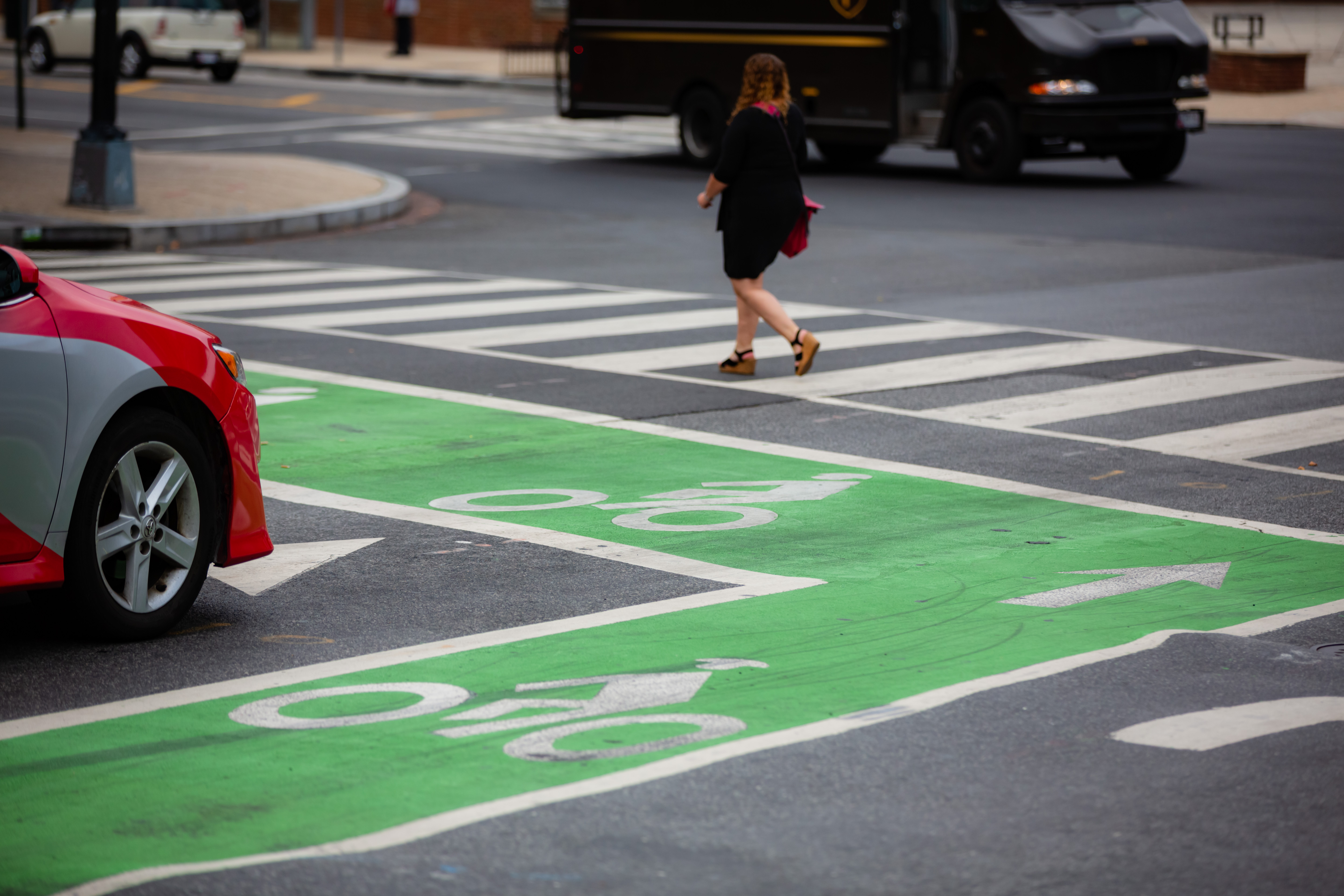The photograph captures a dynamic city street scene centered around a crosswalk marked in white against a charcoal gray street, accented with green bike lanes. A red and gray car has halted at the intersection, waiting for a woman who is mid-crosswalk. She is adorned in a black dress with a red collar, high-heeled shoes, and carries a pink purse. Her long, tannish hair flows down as she faces away from the camera. To her right looms a large black and silver UPS truck with distinctive UPS lettering, positioned perpendicularly to her movement. In the background, on her side of the street, a white SUV is parked along the curb, completing the bustling urban tableau.